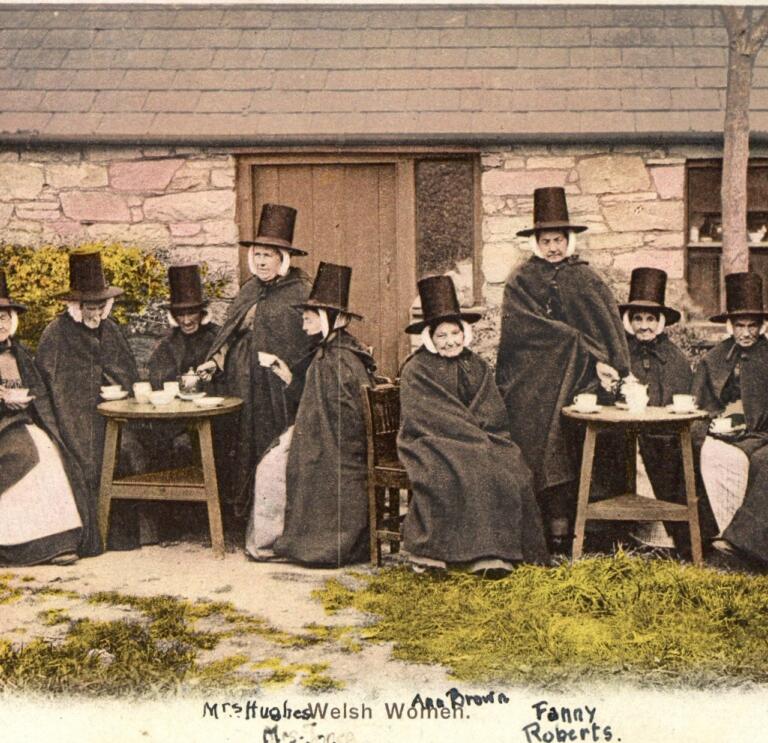This black-and-white photograph features a group of people, both men and women, seated and standing around small tables outside a stone cottage with a wooden door. The people are dressed in long shawls and cloaks with hoods, reminiscent of period attire, and most are wearing stovepipe hats. On the tables, there are white coffee cups and a small metal silver tea kettle, suggesting they are enjoying a tea gathering. The scene is set on patches of grass, with a green hedge on the left and a tree on the right near a window of the house. The photograph, titled "Mrs. Hughes Welsh Women, Anna Browna, Fanny Roberts," includes a total of nine people—seven seated and two standing—capturing a moment of historical reenactment with the individuals displaying a range of expressions, from stern to neutral.